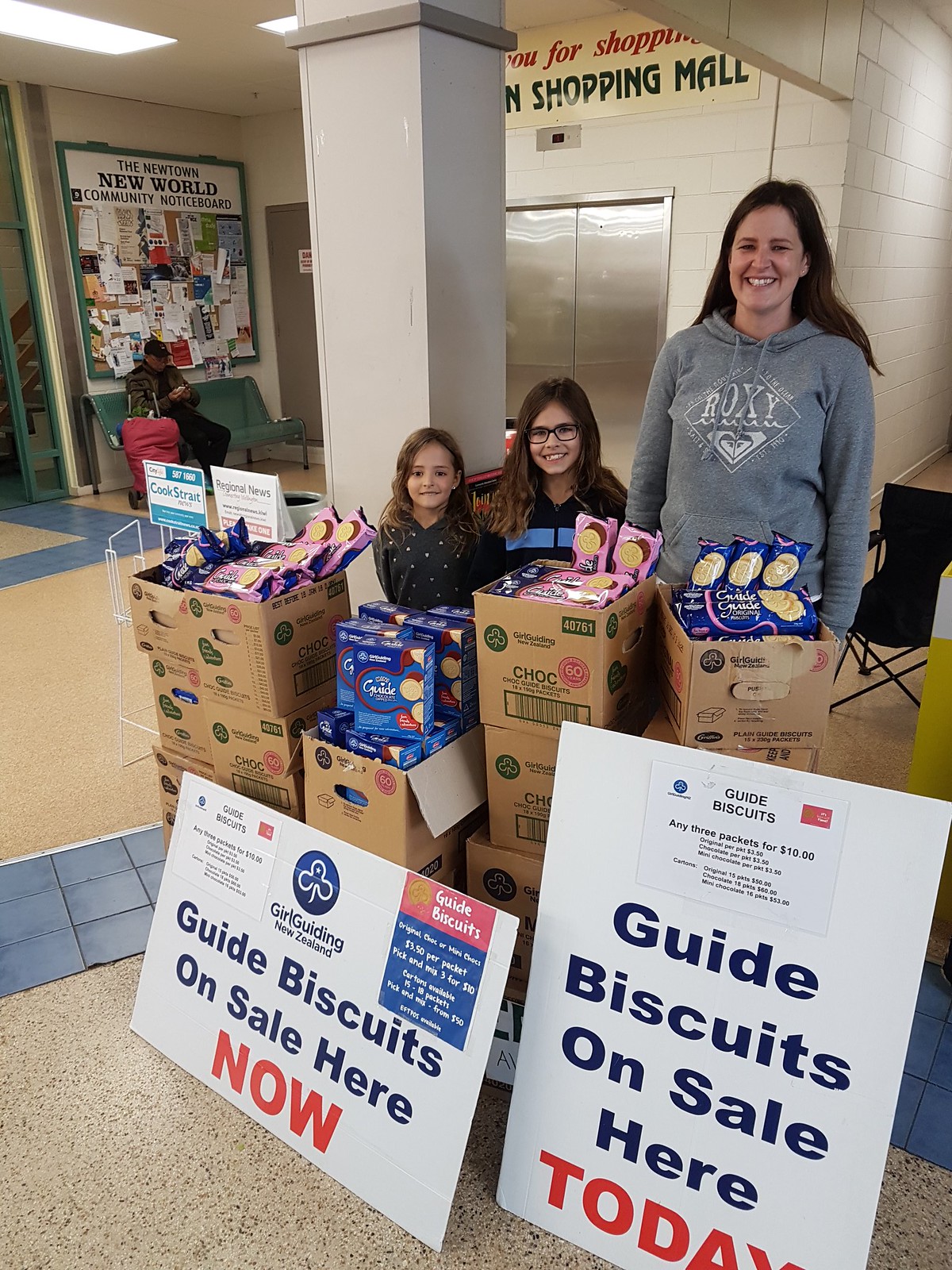In the image, three Caucasian females, likely a mother in her late 20s and her two children, are standing prominently behind several boxes of Girl Guide cookies. The boxes are brown and display various styles of biscuits, specifically four different kinds. In front of the boxes, there are two white signs with the phrases "Guide biscuits on sale here now" and "Guide biscuits on sale here today." Additionally, pricing details indicate options such as any three packets for $10, individual packets at $3.50 each, and bulk packages.

The group is positioned near a white pillar inside what appears to be a shopping mall, evidenced by a sign in the background over a silver elevator that reads "Thank you for shopping" with "shopping mall" in black letters beneath it. To the left of the pillar, a person is seated on a green bench with a red bag and is looking at their phone, in front of a bulletin board labeled "The Newtown New World Community Notice Board."

This well-detailed scene captures the lively atmosphere of a shopping mall where cookies are being sold, possibly for a fundraiser or community event.